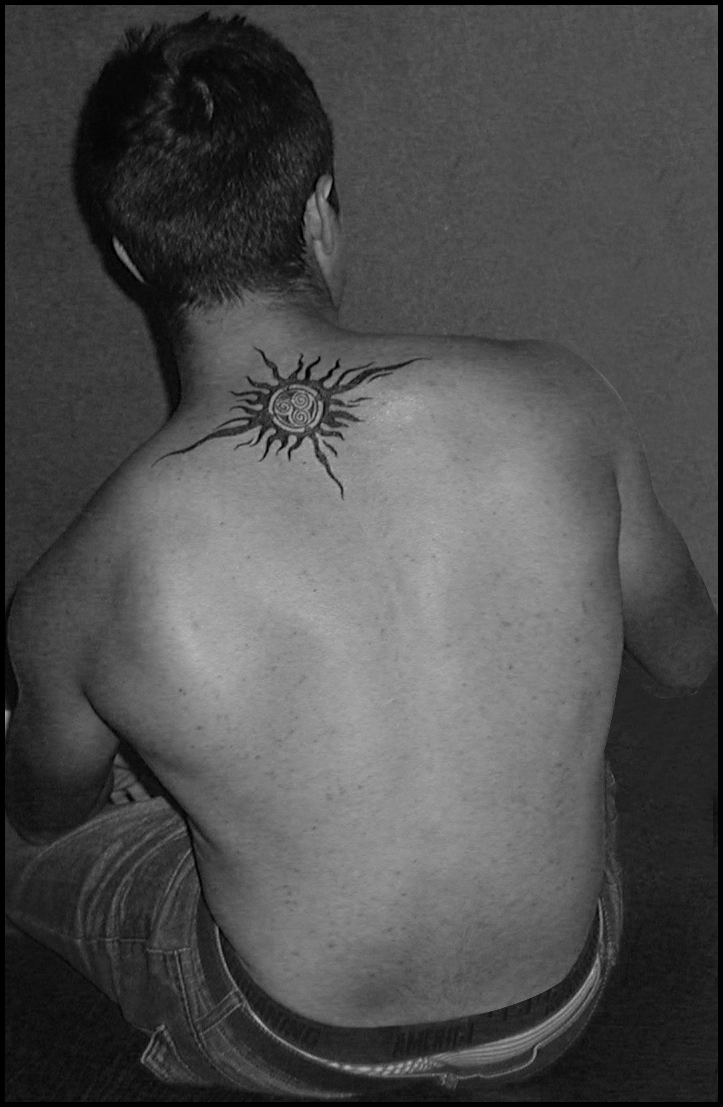A black and white photograph captures a shirtless Caucasian man sitting with his back to the camera. His short, dark hair neatly frames the top of his head, which is positioned in a way that his face remains unseen. Between his shoulder blades, prominently displayed, is an extensive tattoo resembling a sunburst with intricate, swirly designs at its center. The tattoo's rays radiate symmetrically across his shoulders, extending partway down his back. His muscular build is juxtaposed with the casual attire of slightly sagging jeans, revealing the waistband of his underwear. He sits in a contemplative pose with one hand resting on his knee, facing a gray wall which contrasts against the black bottom of the photograph, emphasizing the stark, artistic qualities of the image.